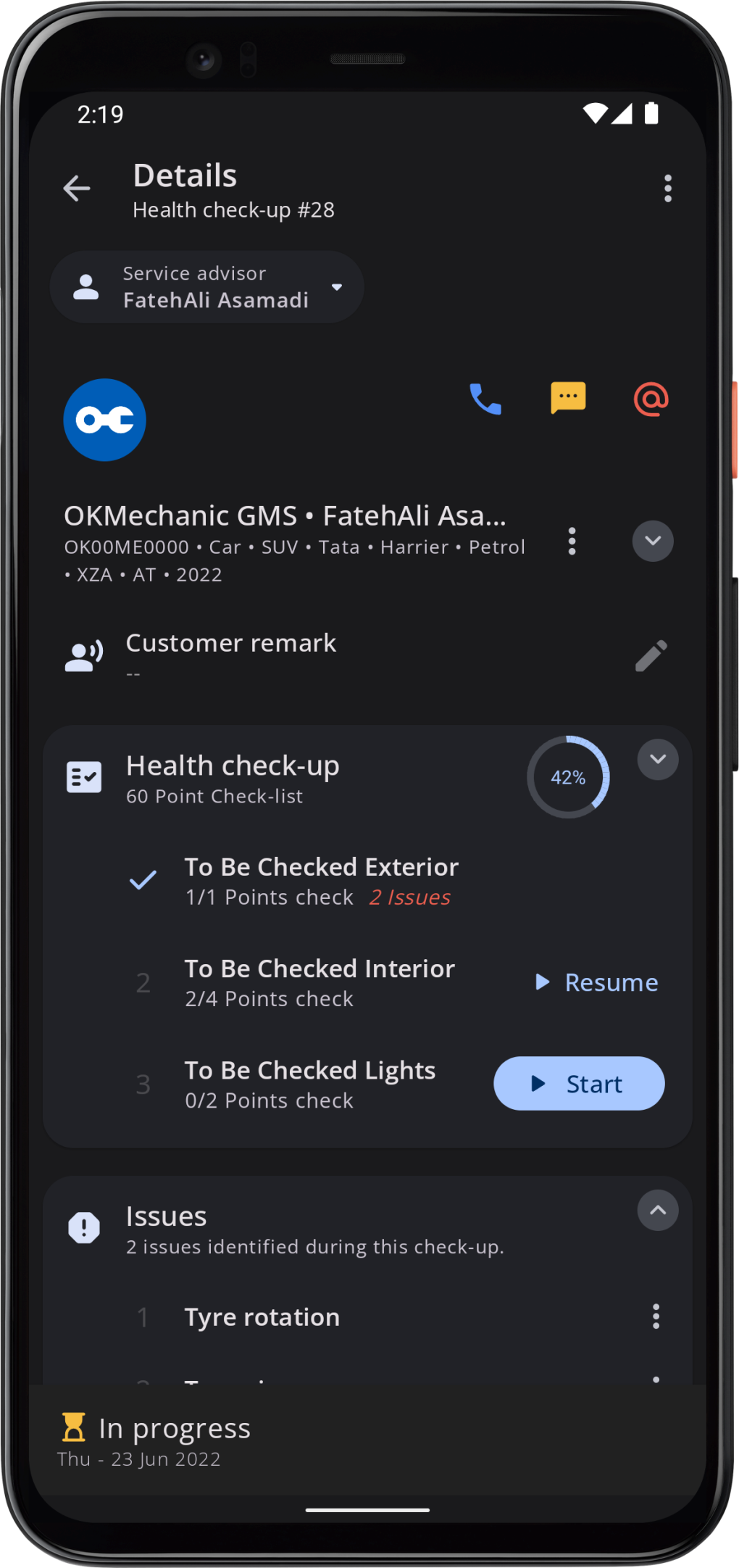This is a detailed and polished caption based on the voice description provided:

---
The graphic showcases a smartphone with a black bezel at the top, where the selfie camera lens and a small gray dash are visible. The screen has been digitally manipulated to display a mock interface. The background of the screen is black with white font. At the top, the time is shown as 2:19, accompanied by icons representing full WiFi, full mobile signal, and a full battery—these icons are artificially added for effect. 

Below this status bar, the text reads: "Details, Health Checkup, Number 28, Service Advisor, Fatah Ali Asmadi." Following this, there is a blue circle containing a white wrench symbol, next to which are icons depicting a blue phone, a yellow chat bubble, and a green @ symbol. Further down, the screen displays: "OK Mechanic, GMS, Fatah Ali Asmadi." The final line of text reads: "OK00ME000.car.suv.tata.harrier.petrol.xza.at.2022."
---

This caption provides a comprehensive and detailed description of the graphic.